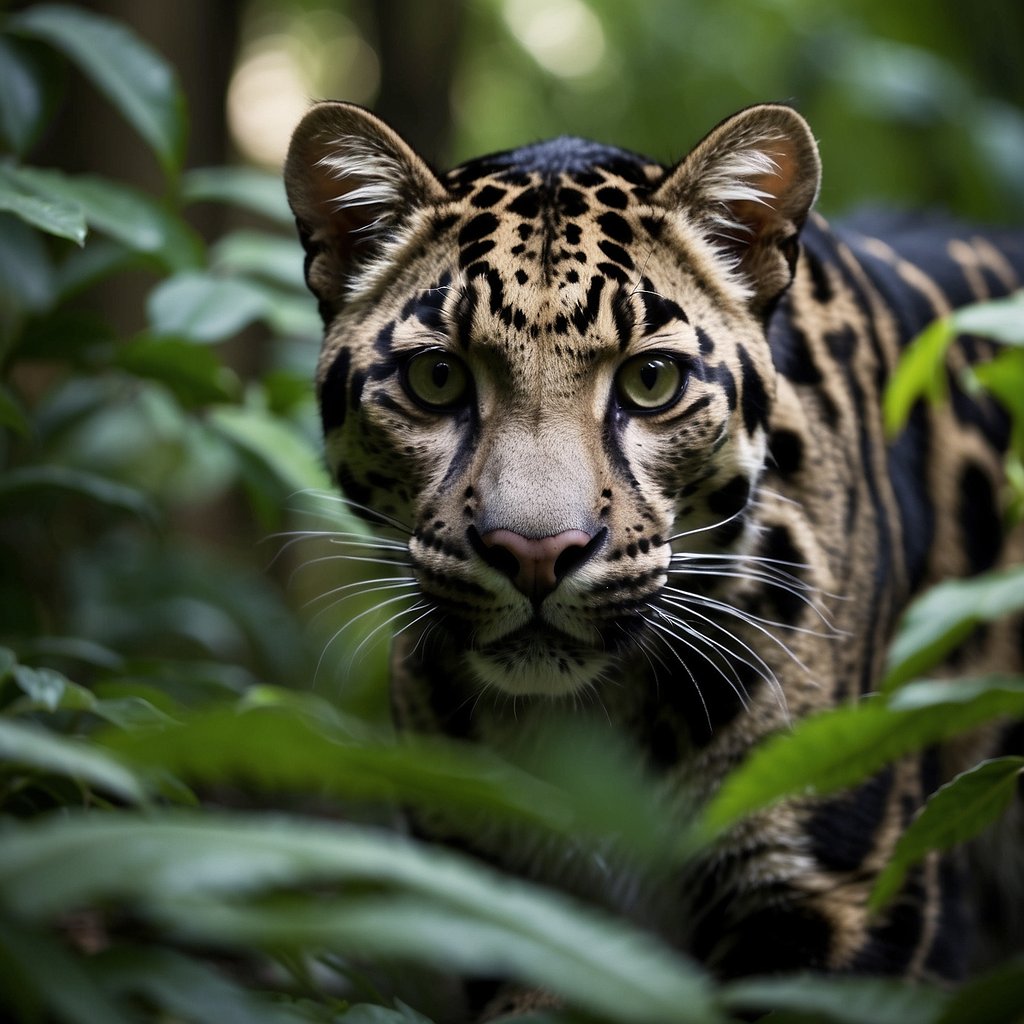This detailed color photograph captures a large wild cat, potentially a leopard, jaguar, or cheetah, characterized by its tan fur adorned with black spots and stripes. The cat's intense yellow-green eyes are fixed directly on the camera, giving the image a powerful, direct gaze. The cat features prominent white whiskers and a pinkish nose. Surrounding the cat are lush, dark green leaves, with long plant fronds partially obscuring its body, giving a sense of the animal stealthily navigating through dense foliage. The background is intentionally blurred, ensuring that the focus remains on the cat’s strikingly clear visage. The captivating and mysterious nature scene includes no other animals, people, text, or structures, emphasizing the solitary majesty of this wild predator.